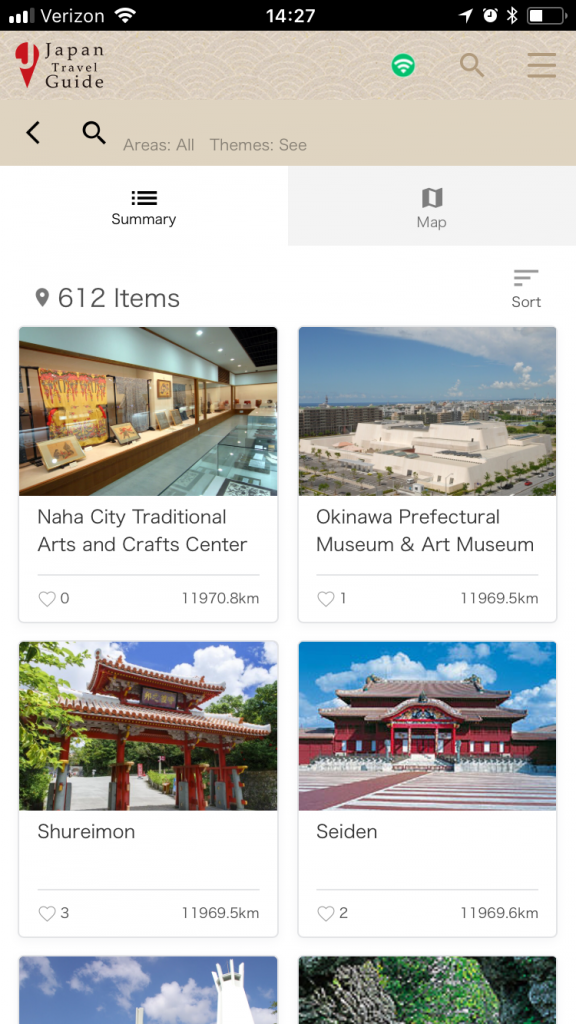The image features a white background at the very top and prominently displays a black bar with the Verizon logo and the number 1427. Below the black bar, there is a purple header box with a small red icon containing a "J" symbolizing Japan Travel Guide. Beside it, there is a green circle with three horizontal lines and a magnifying glass icon, along with an additional set of three straight lines followed by a left-facing arrow and another magnifying glass. This section is labeled with "areas" and "all themes". 

Following this, the interface includes a white summary button with three bulleted lines and dots, a blue map button, and a gray pointer icon indicating "612 items". Another section with three lines labeled "sort" is present. The content below this section lists several places of interest:

- **Neha City Traditional Arts and Crafts Center**: Zero hearts, 11,970.8 KM away.
- **Okinawa Prefectural Museum and Art Museum**: One heart, 11,969.5 KM away.
- **Shuriman**: Three hearts, 11,969.5 KM away.
- **Sidon**: Two hearts, 11,969.6 KM away.

The image concludes with two additional pictures that are partially cut off.